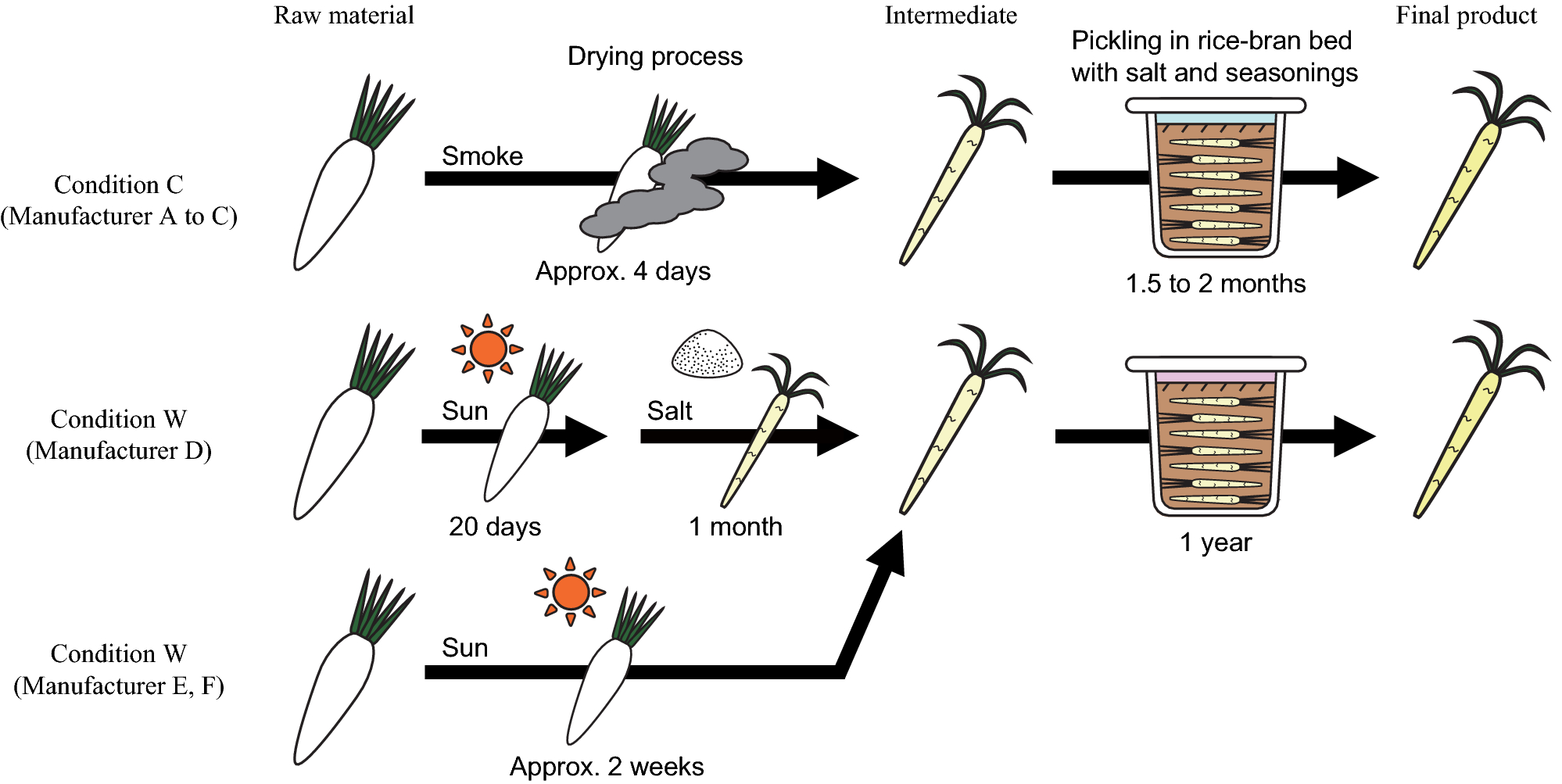The image depicts a detailed flowchart illustrating the transformation of raw vegetables, specifically carrots, through various processing conditions to create a final pickled product. The process begins with the raw material, which undergoes different drying methods based on the specified conditions. 

**Condition C** (Manufacture A to C) involves a drying process using smoke for approximately four days, resulting in an intermediate product that is then placed into a rice bran bed for pickling with salt and seasonings, a stage lasting 1.5 to 2 months.

**Condition W** ([Manufacture D](there is only one W mentioned, but two conditions. D, E, F are grouped under the 'W') involves two distinct drying stages: sun exposure for 20 days followed by salting for one month, leading to an intermediate product. This intermediate product undergoes pickling in a rice bran bed with salt and seasonings for one year.

Another instance of **Condition W** (Manufacture E and F) describes an initial sun drying process lasting two weeks. This product then combines with the salted intermediate from the previous process before undergoing the same pickling in rice bran bed with salt and seasonings.

After each condition-specific drying and pickling regimen, the final product is a yellow, pickled carrot, visually distinct from the initial raw material. The chart meticulously outlines the timeframe and specific steps involved in transforming the vegetables from raw material to the final, seasoned, pickled product.